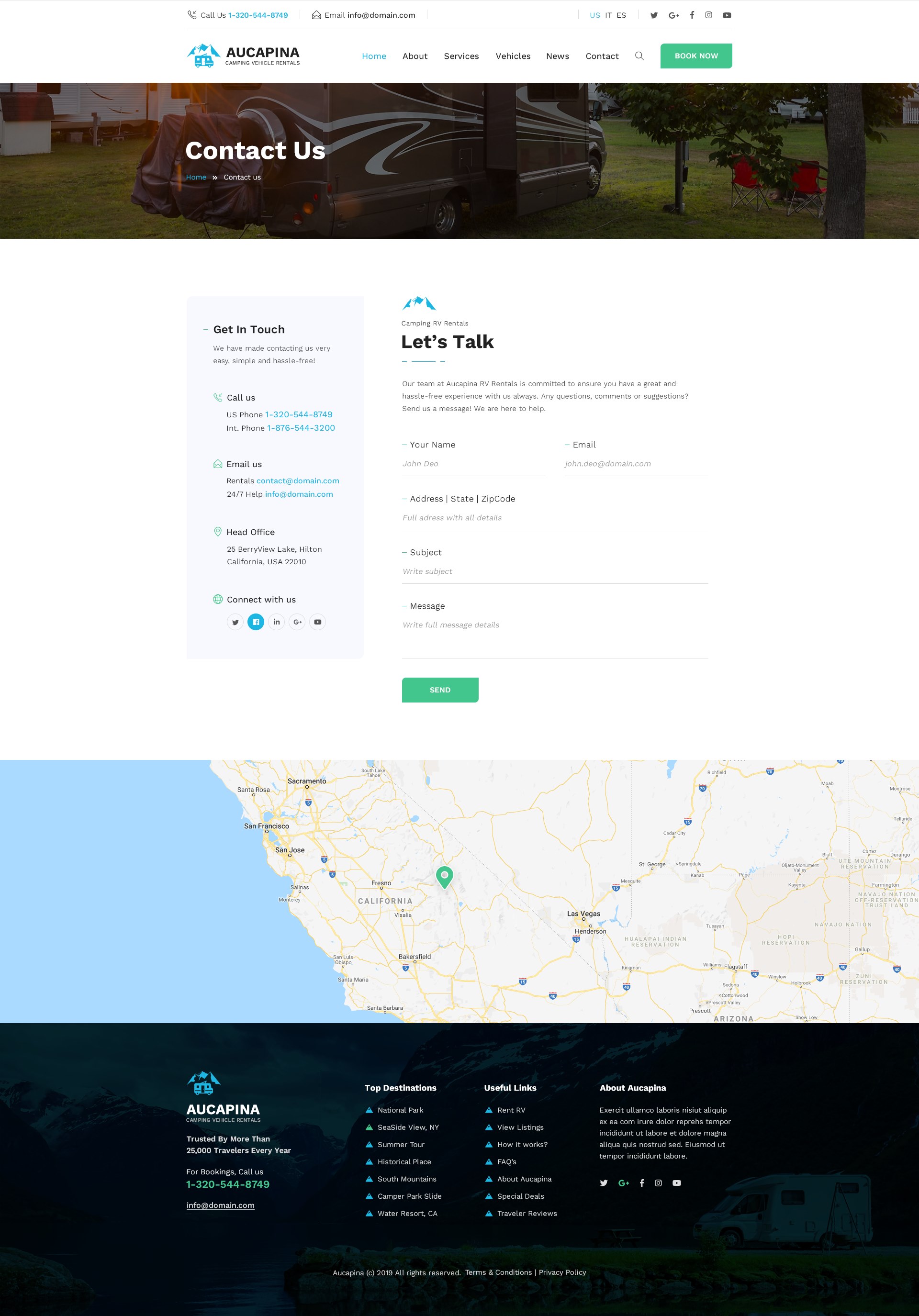This screenshot captures the contact page of the Alcapina website, a potential vehicle or RV rental service. Due to the small and blurry text, the words are difficult to decipher even when zoomed in, but key elements can be identified.

At the top of the page, the header reads "Contact Us," accompanied by a green "Book Now" button to the right. The horizontal navigation menu includes options for Home, About, Services, Vehicles, an unreadable section, and Contact. This suggests the website might specialize in vehicle rentals, particularly RVs, as indicated by the background image of an RV behind the "Contact Us" header.

Below the main header, a grey box titled "Get in Touch" provides fields for phone numbers, email, and the head office location, along with possible links to social media profiles. To the right of this box, another section labeled "Let's Talk" (potentially with a tagline like "Camping for America") offers a contact form requesting the user's name, email address, subject, and message.

The lower part of the page features a partial map of California, possibly indicating the primary service area of Alcapina. At the bottom of the screen, a large black footer likely includes standard webpage information such as details about the company, FAQs, and additional resource links, though the text is not readable.